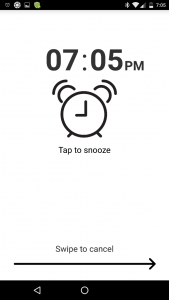This image is a screenshot from a cell phone captured at 7:05 PM. At the top of the screen, there is a slightly blurry black status bar featuring various icons. On the left, a discernible settings icon is visible along with a green bubble icon that is too blurry to identify clearly. On the right side, icons for Bluetooth, Wi-Fi (showing two bars), very low battery status, and the current time, either 7:05 or 7:06, are displayed.

Directly below this status bar, the time "7:05 PM" is prominently displayed in a large, bold font, ensuring clear legibility despite the blurriness. Beneath the time, there's an old-school alarm clock icon with a round body. The icon features legs diagonally positioned to the left and right and small half circles at the 11 o'clock and 1 o'clock positions to represent metal bells. The alarm is set to 9 o'clock and includes a "Tap to snooze" instruction.

At the bottom of the screen, in black text, there's the message "Swipe to cancel" accompanied by a lengthy black arrow pointing to the right. Just below this, a black bar is present, which houses a left-facing triangle on the left side and a white circle in the center, while the right side remains empty.

The overall composition of the screenshot captures a moment in time on a cell phone's interface, highlighting crucial elements such as the time, an active alarm, and navigation instructions.